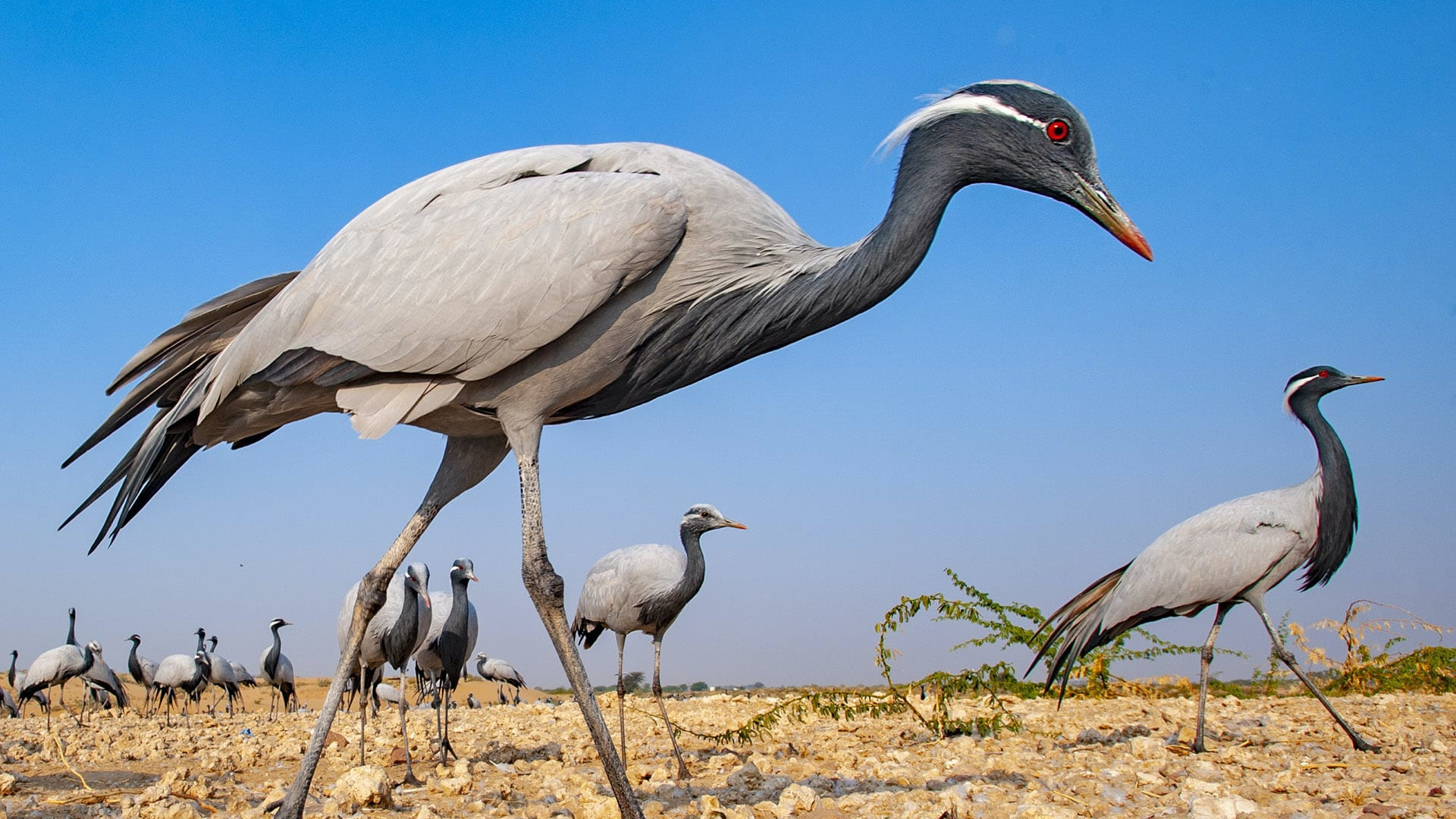The image is a striking wildlife photograph featuring a close-up of a large bird in the foreground, with a backdrop of numerous similar birds. The prominent bird in the foreground, identified as a heron, stands on rocky, dry, light brown ground interspersed with shallow water and patches of greenery. This heron has a predominantly grey body, black feathers on its neck and head, vivid red eyes, and a red-tipped beak. Its tail feathers are dark brown and black, and it stands on long, thin legs. There are approximately twenty other birds in the background, sharing similar characteristics but appearing slightly smaller due to their distance from the camera. Although they all vary in position and orientation, the overall scene is set against a bright blue sky, highlighting the rugged terrain and the detailed features of these impressive birds.